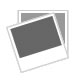The photograph captures a large ring, comparable in size to a class ring, set against a plain white backdrop, suggesting a focus solely on the ring itself—likely fit for an advertisement. Central to the ring is a striking gem, described variably as a purplish or pinkish jewel, giving off an aura that teeters between an emerald and a ruby. This gem is encased in a black setting interwoven with silver lines, lending it an intricate yet sturdy appearance.

Prominent in the design are three silver balls or dots situated around the jewel, further complemented by a silver rim encircling the gem, which itself is accentuated by a glass-like covering. The ring's band diverges into a detailed design that seems partially obscured by shadows or angle, hinting at rope-like patterns and possible signs of wear or rust along the edges. This sophisticated piece, possibly crafted from sterling silver or bronze, is photographed at a 45-degree angle, highlighting both the jewel and the nuanced craftsmanship of the ring.